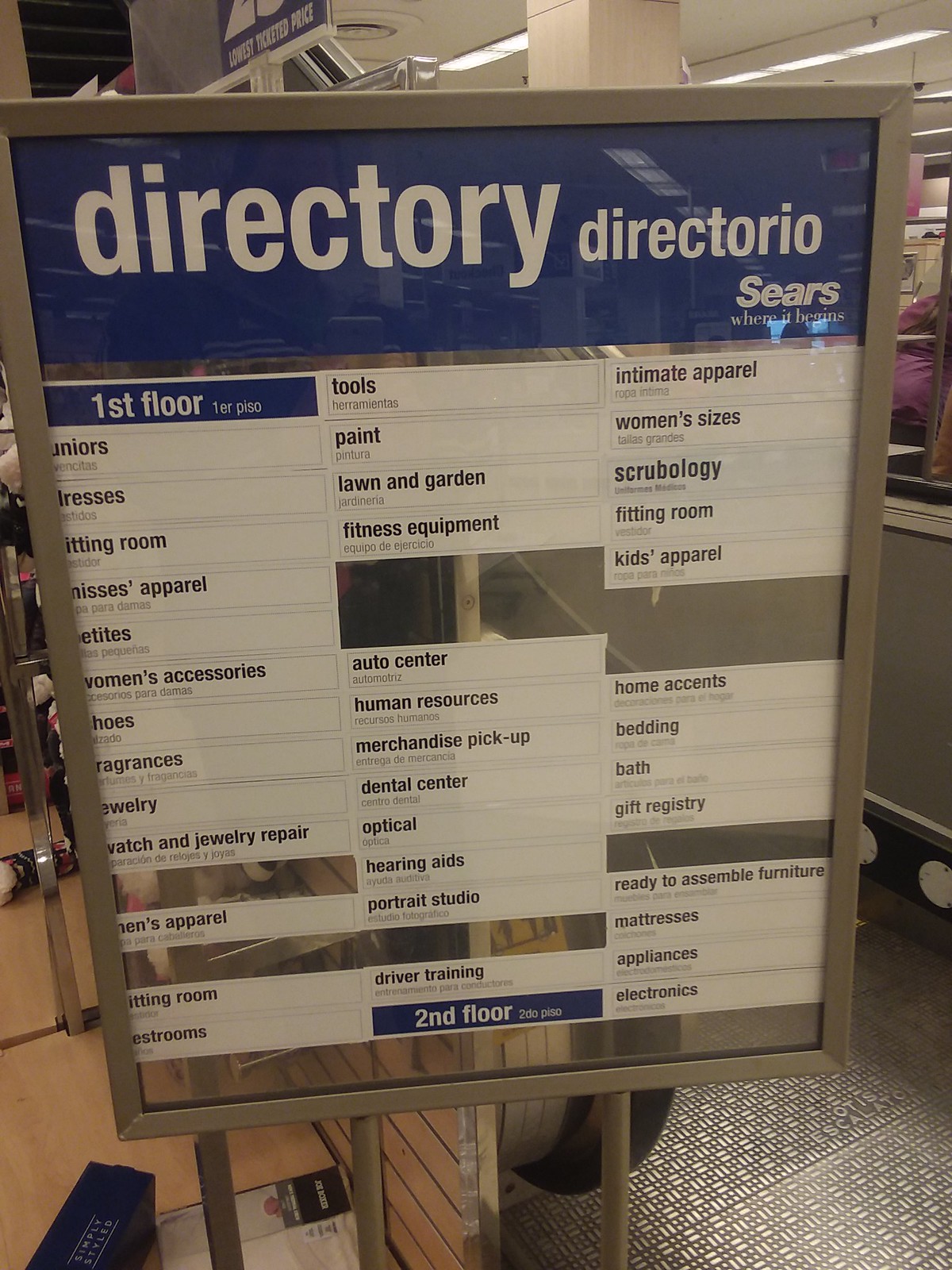This image captures a retail shop's directory board, detailing the various facilities available on each floor of the building. The first floor features sections for juniors, dresses, fitting rooms, apparel, women's accessories, and fragrances. The second floor is designated for tools, painting supplies, intimate apparel, and a section presumably for scrubology. Notably, parts of the directory are omitted and missing. The directory board itself is mounted on a wooden and metal fixture, which is suspended beside a set of escalators with an aluminum base.